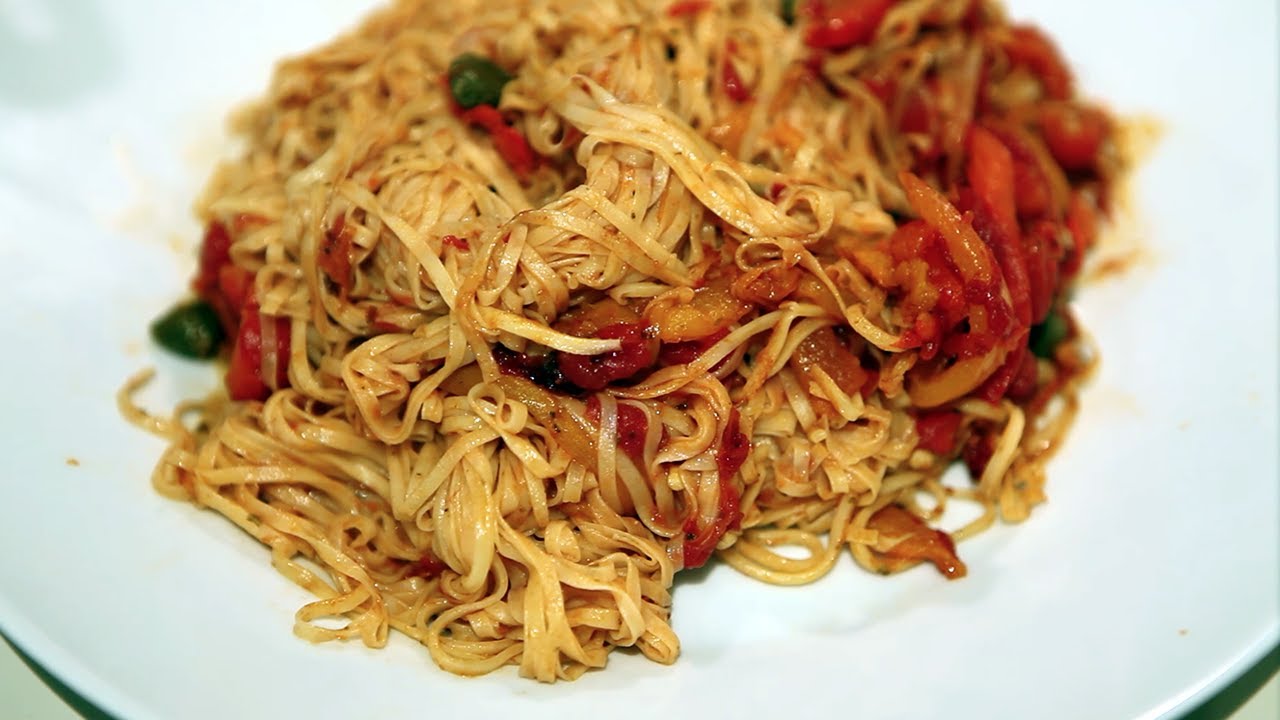This close-up photograph features a white dinner plate with a green trim along the edge, showcasing a dish of fettuccine flat noodles. The noodles have a yellow-golden hue and are richly coated with a red tomato sauce that appears to have been thoroughly mixed throughout. This sauce contains a variety of minced and chopped vegetables, and scattered chunks of ingredients such as possibly chicken, tomatoes, and olives. The dish is presented in a pile, with some olives and tomato pieces more visibly sticking out on the sides. The image sharpens on the forefront details of the pasta while the background softly blurs, emphasizing the texture and overall vibrant, red-tinted presentation of the meal. The plate is positioned prominently, with only the bottom and right corners of the table faintly visible.